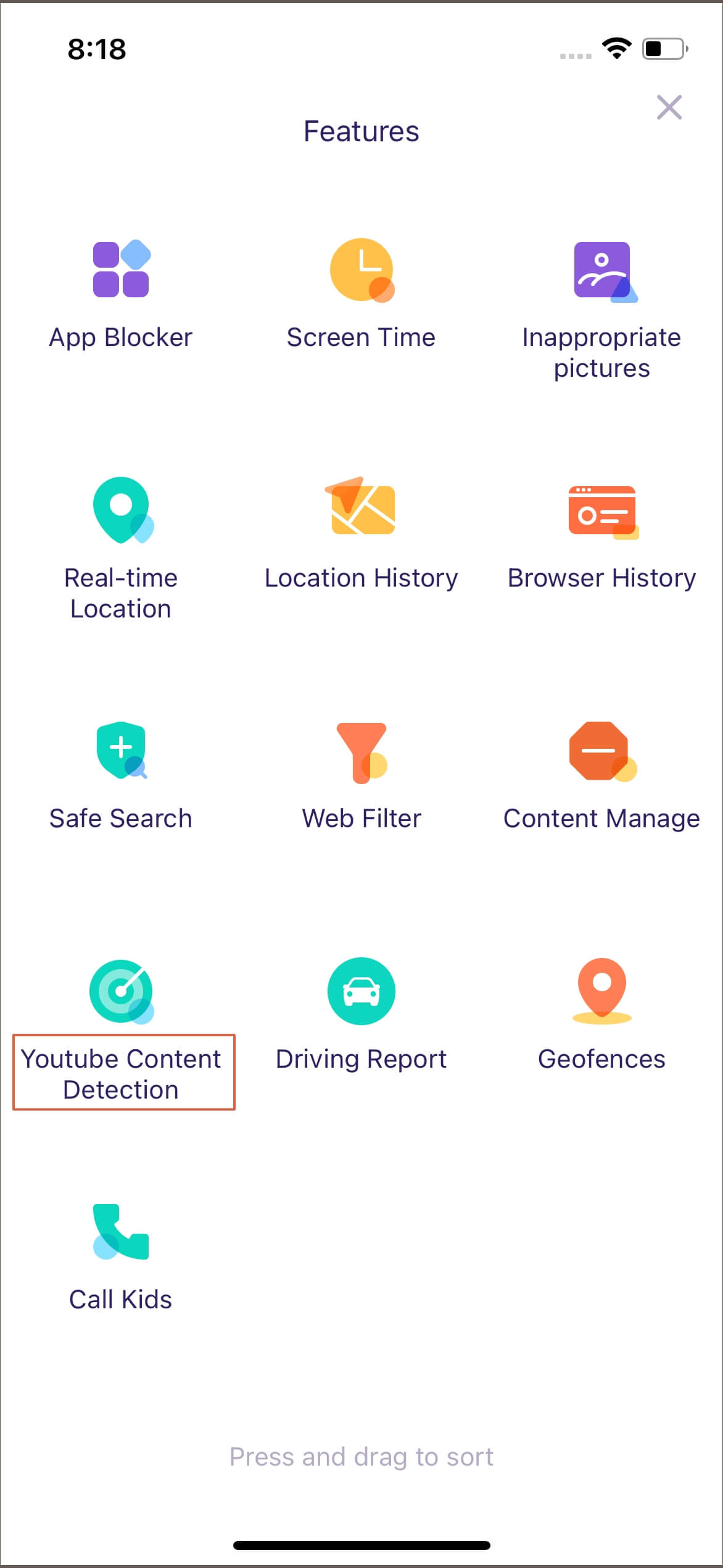A screenshot of a mobile phone screen with a white background. At the top left corner, the time is displayed as 8:18 in black font. The top right corner features four small gray horizontal dots, indicating settings or a menu, along with full Wi-Fi bars and a half-charged battery icon. Below the status bar, a menu labeled "Features" is open, with a small gray ‘X’ next to it for closing the menu.

The menu lists five rows of three features each, in a grid format:

1. **App Walker**: Represented by an icon of three cubes, with one turned sideways.
2. **Screen Time**: Illustrated by a yellow clock icon.
3. **Inappropriate Pictures**: Depicted with a photo icon.

4. **Real Time Location**: Marked by a location bubble icon.
5. **Location History**: Shown with a map icon.
6. **Browser History**: Illustrated with a credit card icon.

7. **Safe Search**: Represented by a shield with a cross icon.
8. **Web Filter**: Illustrated with a flashlight icon.
9. **Content Manage**: Depicted with a stop sign icon.

10. **YouTube Content Detection**: Highlighted in red, without an explicitly described icon.